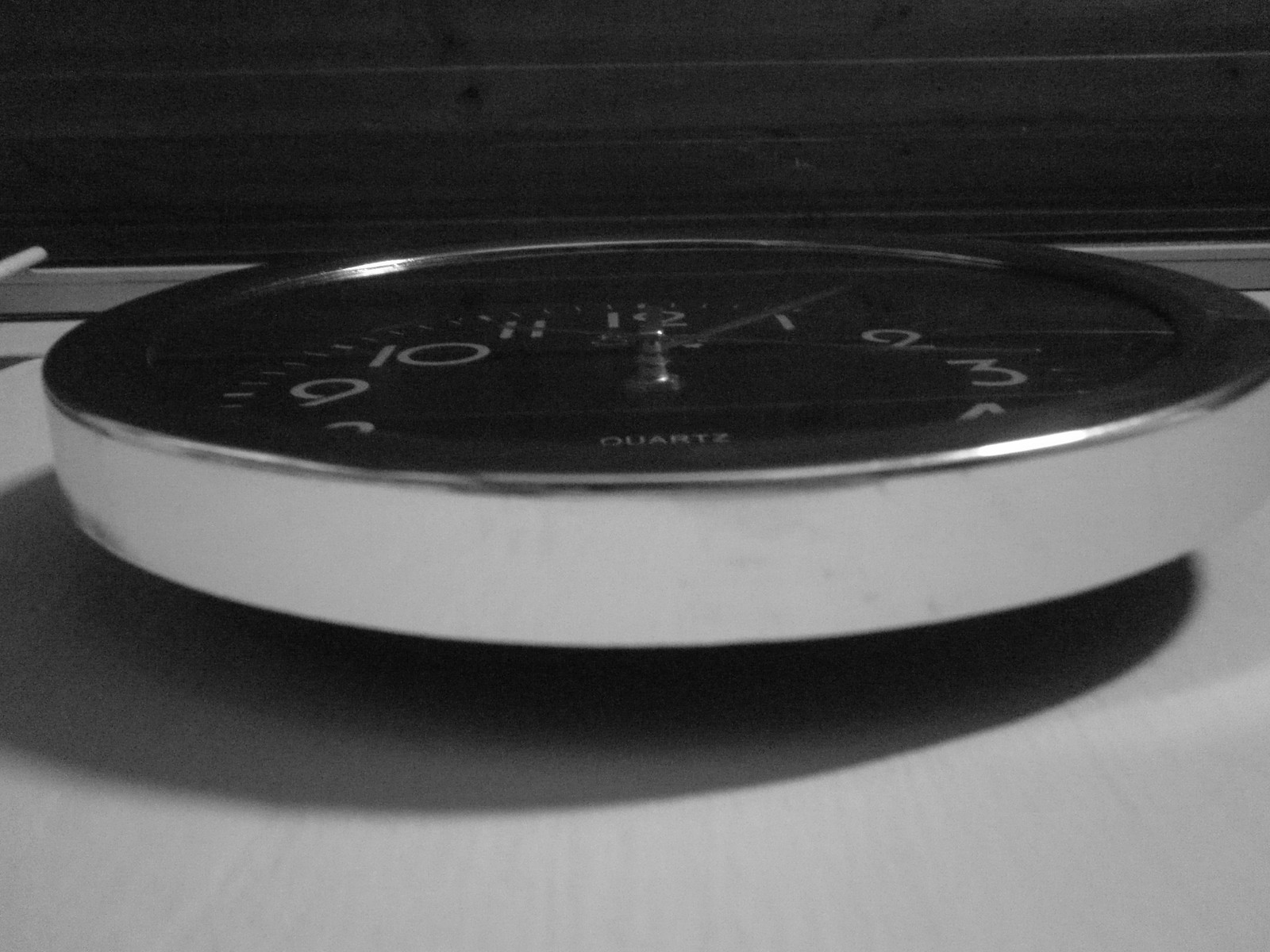This image depicts a clock viewed from an unconventional angle, seemingly from underneath. The clock casts a distinct shadow on the surface behind it, indicating that a light source is positioned overhead. The top of the clock reflects this light, creating two visible shiny marks. The clock itself appears predominantly metallic, with a silver side that looks reflective. Due to the perspective, the front edge of the clock appears darker, either due to the angle or the actual coloring.

The clock face is black, accented by white numerals in a basic, legible font. The hands of the clock are silver; however, the presence of a second hand is indiscernible from this vantage point. The background, presumably the ceiling above the clock, is dark with occasional spots that could be small holes or imperfections. This composition creates a dramatic and somewhat mysterious atmosphere, highlighting the interplay between light, shadow, and metallic surfaces.